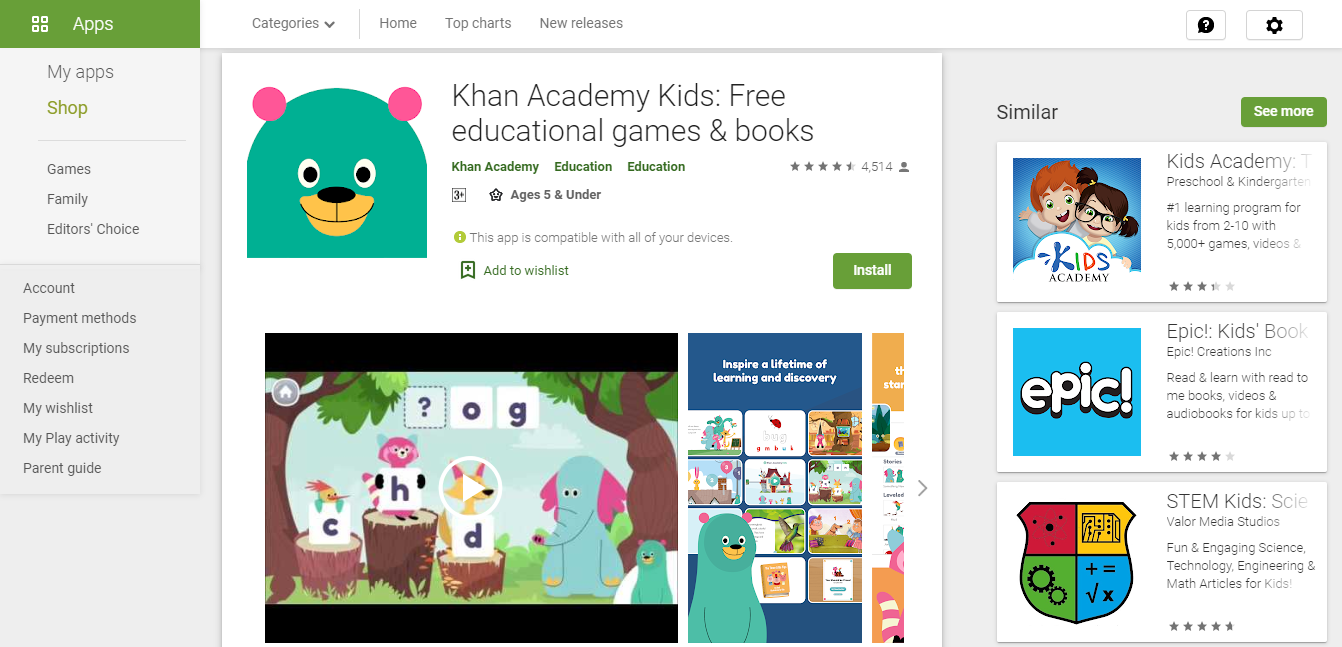**Caption:**

The image appears to be a screenshot from the Google Play Store. In the upper left-hand corner, there is a green background with the word "Apps" written on it, followed by a grey bar featuring options like "My apps" and "Shop". Below this, smaller text lists categories such as "Games", "Family", "Editor's Choice", among others.

On the left side, there are options for "Account", "Payment methods", "My subscriptions", "My wishlist", "My play activity", and "Parent guide". At the upper center of the screen, categories such as "Home", "Top charts", and "New releases" are visible.

The focus of the page is on the "Khan Academy Kids" app, which falls under free educational games and books. It is targeted towards children aged 5 and over. The icon for the app is a cartoon bear's head with a green face, a yellow snout, a smiling mouth, and pink ears. A green "Install" button suggests that the app is compatible with all devices.

Underneath, there are various screenshots from the app: one depicts animals in a woodland setting holding up letters, another shows an elephant, and more preview pages are aligned to the right. To the far right, the section labeled "Similar" showcases related apps: "Kids Academy: Preschool and Kindergarten" featuring a picture of two kids, "EPIC Kids Books and Educational Games" with "EPIC" written in white on a blue background, and a STEM-related kids' science app adorned with a colorful crest displaying math and science symbols.